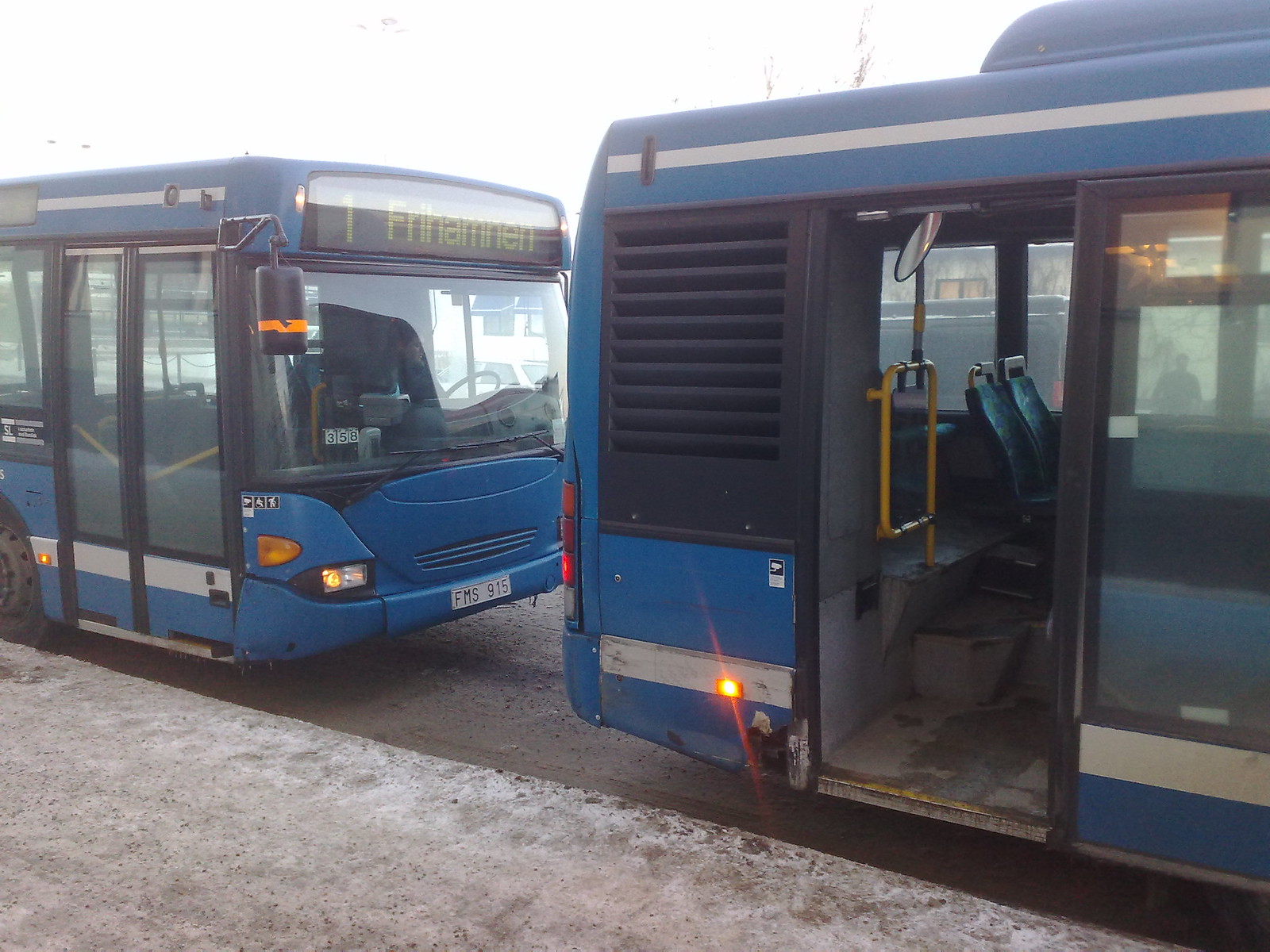The image captures a scene of two blue public buses with light gray horizontal stripes parked at a curb. The bus on the left displays the front part with its headlights on and a license plate reading FMS 915, although the issuing jurisdiction is not legible. The bus on the right shows the rear, with its red marker light illuminated and the back door open, revealing a metal yellow railing and blue seats with a gray floor. Both buses feature black trim around the windows and doors, and have a flat front with a wide windshield. Overcast sky lends a grayish light to the scene, highlighting the weathered gray sidewalk with dark spots and the pebbly, churned gray road. Visible through the bus windows are faint branches of a brown tree, a building, some vehicles, and a few pedestrians. The front bus has a destination sign at the top, partially readable as "Free Homnin."